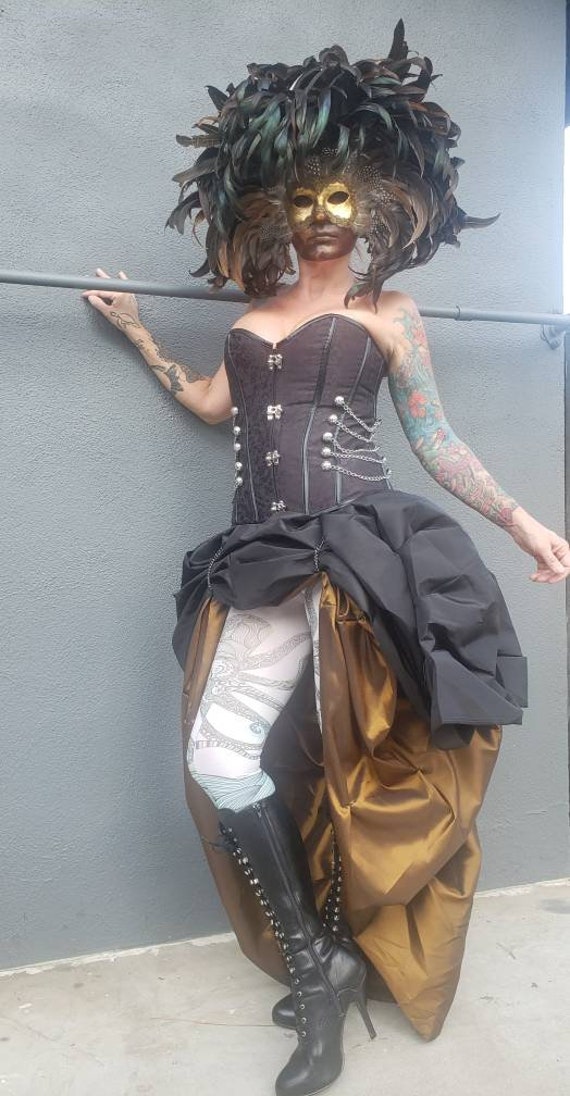In the photograph, a woman dressed in a striking costume stands against a gray wall, her hand resting on a nearby gray pipe. She wears an elaborate black corset bustier, adorned with black lace, silver buttons, chains, and black boning down the front. Her black satin skirt is pulled up in the front, revealing a gold underlayer that's also hitched up, and white stockings featuring an octopus design on the thigh. Completing her outfit, she has on high-heeled, black leather knee-high boots with silver buttons running from top to bottom. Her arms are decorated with tattoos: her left arm displaying a colorful floral sleeve including purple, blue, and red flowers, while her right arm has isolated black designs, such as a headdress, a bow and arrow, and other indistinct motifs. Her face is painted black and she dons a gold mask adorned with dark green feathers and possible pheasant feathers near her face, giving her hair a wild, Medusa-like appearance. The entire scene is set against a darker gray wall contrasting with the lighter gray concrete she stands on.